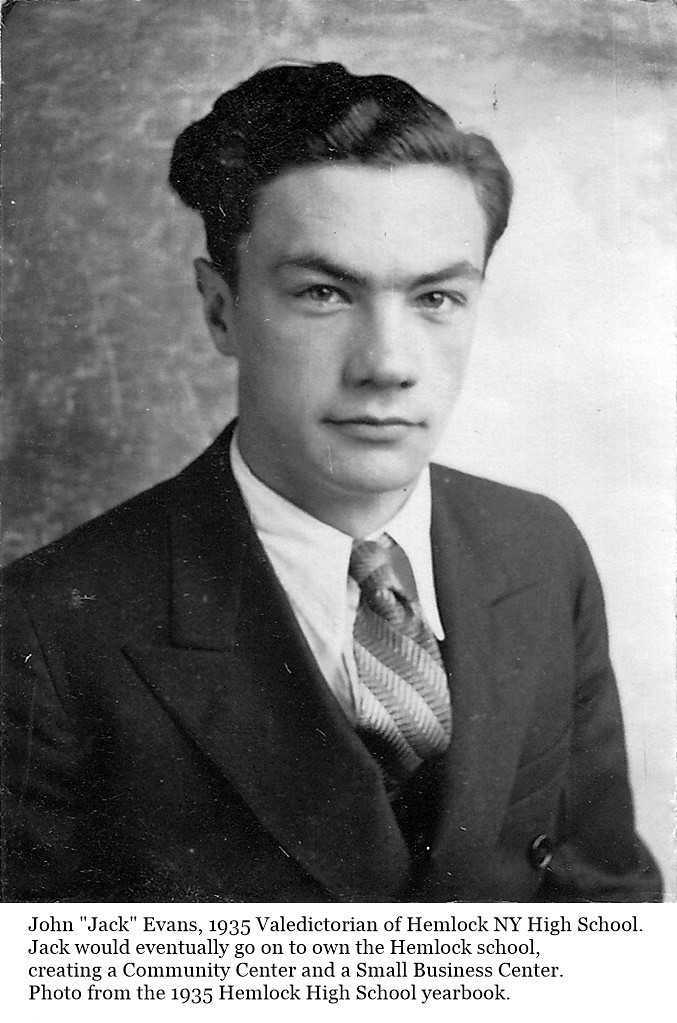The image is a vintage black and white photograph of a Caucasian man named John "Jack" Evans, who was the 1935 valedictorian of Hemlock New York High School. The gentleman, in his 40s, is dressed in a dark-colored suit with a white button-collared shirt and a striped tie, though the actual colors are indeterminable due to the black and white nature of the photo. His hair is black, slicked back, and wavy on top, giving it a puffy appearance at the back. He has dark eyes and eyebrows, and he is posed with a serious expression, lips closed. The background is predominantly white with a slightly darker shade on the left-hand side. The caption at the bottom reads, "John 'Jack' Evans, 1935 valedictorian of Hemlock NY High School. Jack would eventually go on to own the Hemlock School, creating a community center and a small business center." The photograph is from the 1935 Hemlock High School yearbook.